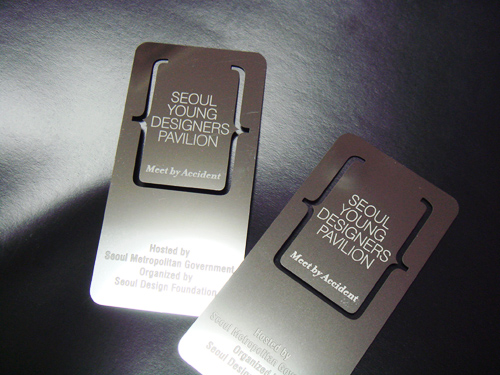This photograph showcases two expertly crafted silver pass cards, which could also be described as premium bookmarks or badges. These cards are elegantly designed with a reflective, metallic finish and a sophisticated cutout pattern. Both cards prominently feature the text "Seoul Young Designers Pavilion" and the phrase "Meet by Accident." Further down, it states that the event is "hosted by the Seoul Metropolitan Government" and "organized by the Seoul Design Foundation." The cards are laid out on a sleek, black surface, resembling either a table or a leather desk pad. The cutout design not only adds to their allure but also hints at their multipurpose use, potentially as mementos for the attendees of this prestigious gathering focused on young talent in the design industry. Although the bottom text is partially obscured, what can be read indicates more details about the event's organization.